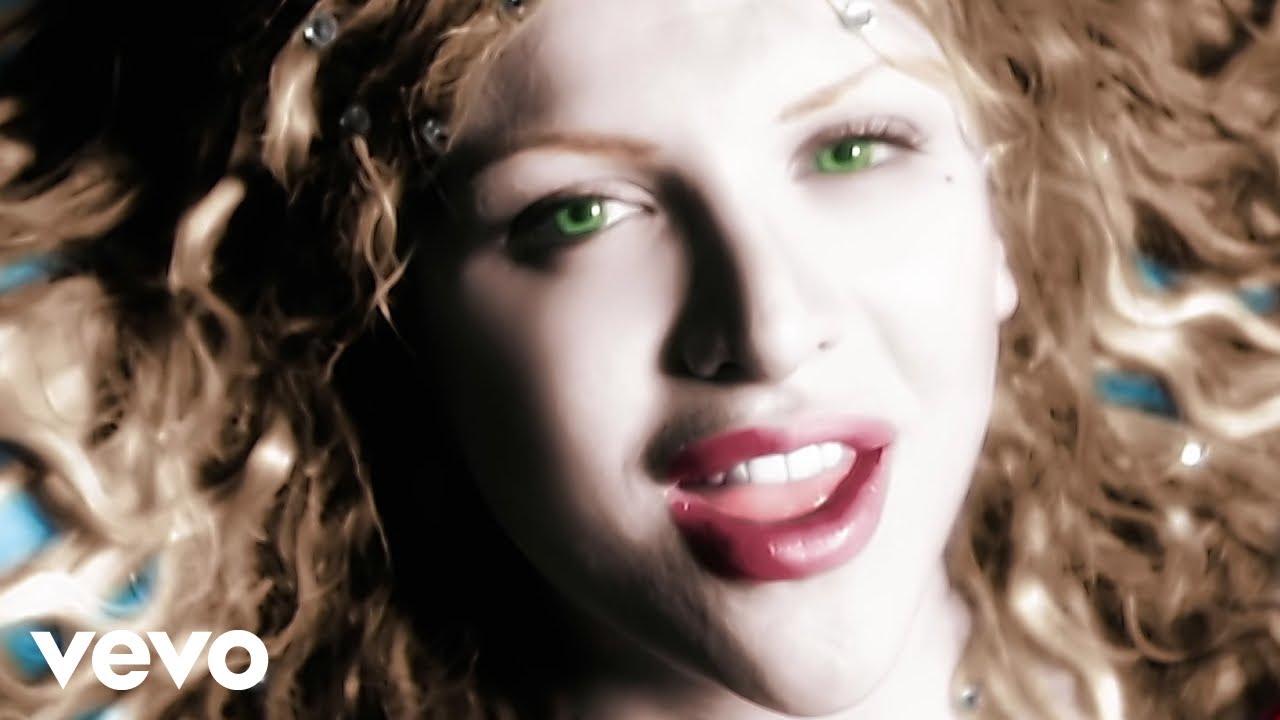The image is a detailed close-up screenshot from the "Celebrity Skin" music video by Hole, featuring Courtney Love. In the shot, Courtney Love's face dominates the frame, extending from her chin to her forehead. She has pale skin with pink lips and her mouth is open as she sings, revealing her white teeth. Her striking green eyes are prominently featured, giving a glowing effect on screen. Courtney's wavy blonde hair surrounds her head, adorned with crystal-like elements that catch the light. She appears to be lying on a blue background, likely the floor of the video set. Notably, the Vevo logo in lowercase white font ('vevo') is situated at the bottom left of the image, indicating the platform on which the video is available.